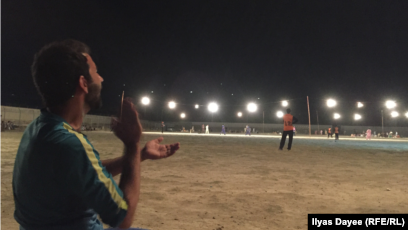The image, taken at night, depicts a vibrant scene at what appears to be a baseball stadium. Captured from behind at approximately five feet away, the main subject is a bearded man with short, dark hair, likely white-skinned, caught in the midst of clapping. He wears a greenish shirt adorned with a white stripe running from the collar to the elbow on his right arm. His right ear is prominently in view. To his right, there are several spectators, some donning orange and black attire, gathered around a field. The field is illuminated by a series of sixteen bright white lights stretching from the man’s clapping hand to the far distance, creating a lively backdrop. The ground near the man is dirt-covered, transitioning to grass further back, with more spectators visible against the night sky. In the bottom right corner of the photo, a black border contains the text "ILYAS DAYEE" followed by "RFE-RL" in parentheses and brackets.